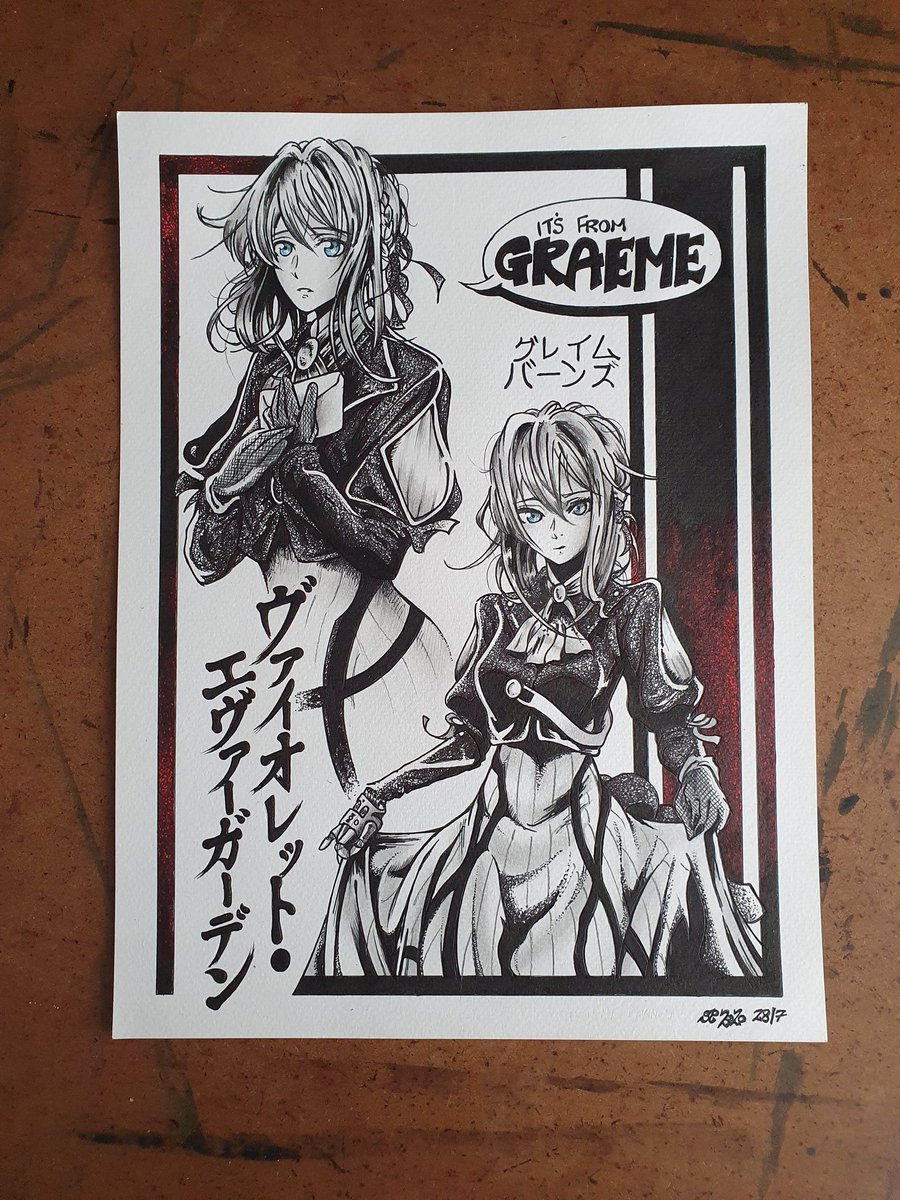The detailed and descriptive caption for the image would be:

"This limited-edition signed print features an intricate anime illustration of two Japanese women with big blue eyes and tousled hair, dressed in elaborate costumes reminiscent of Victorian or cyberpunk styles. Each woman's attire includes long-sleeved, billowing patterned skirts and a neck scarf fastened with a brooch or bow tie. The mostly black and white artwork is accented with splashes of red, creating a striking visual contrast. One woman holds a letter in one pose and her dress in another, while a speech bubble at the top of the image states ‘It’s from Grain.’ The illustration is surrounded by a brown background with deep grey splashes, reinforcing its unique aesthetic. At the bottom right corner, the print is marked with the artist's autograph, date, and edition number, alongside large Japanese characters, highlighting its cultural and artistic value."